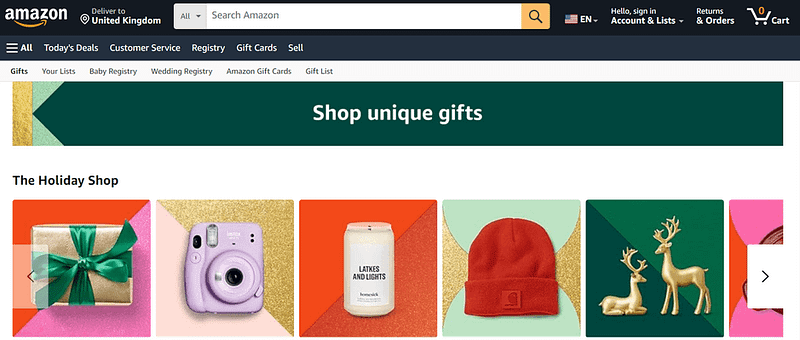The image is a screenshot taken from the Amazon website. In the top left corner, the recognizable Amazon logo is displayed. Adjacent to the logo, on the right, there's a note indicating the website's delivery region as the United Kingdom. Immediately to the right is the search bar with the placeholder text "Search Amazon". Further to the right, the language setting is indicated by an American flag icon accompanied by "EN", denoting English. Next to this is the "Sign-In" button, followed by the "Returns & Orders" button. In the top right corner, a shopping cart icon is visible, showing there are zero items in the cart.

Beneath the main header with the search bar, there are six navigation links: "All," "Today's Deals," "Customer Service," "Registry," "Gift Cards," and "Sell." Below these links, the webpage features a variety of images promoting holiday gifts and Christmas decorations. Among the displayed items are a present wrapped in light gold paper with green ribbons, a camera, an orange beanie, and several deer-themed ornaments or decorations.